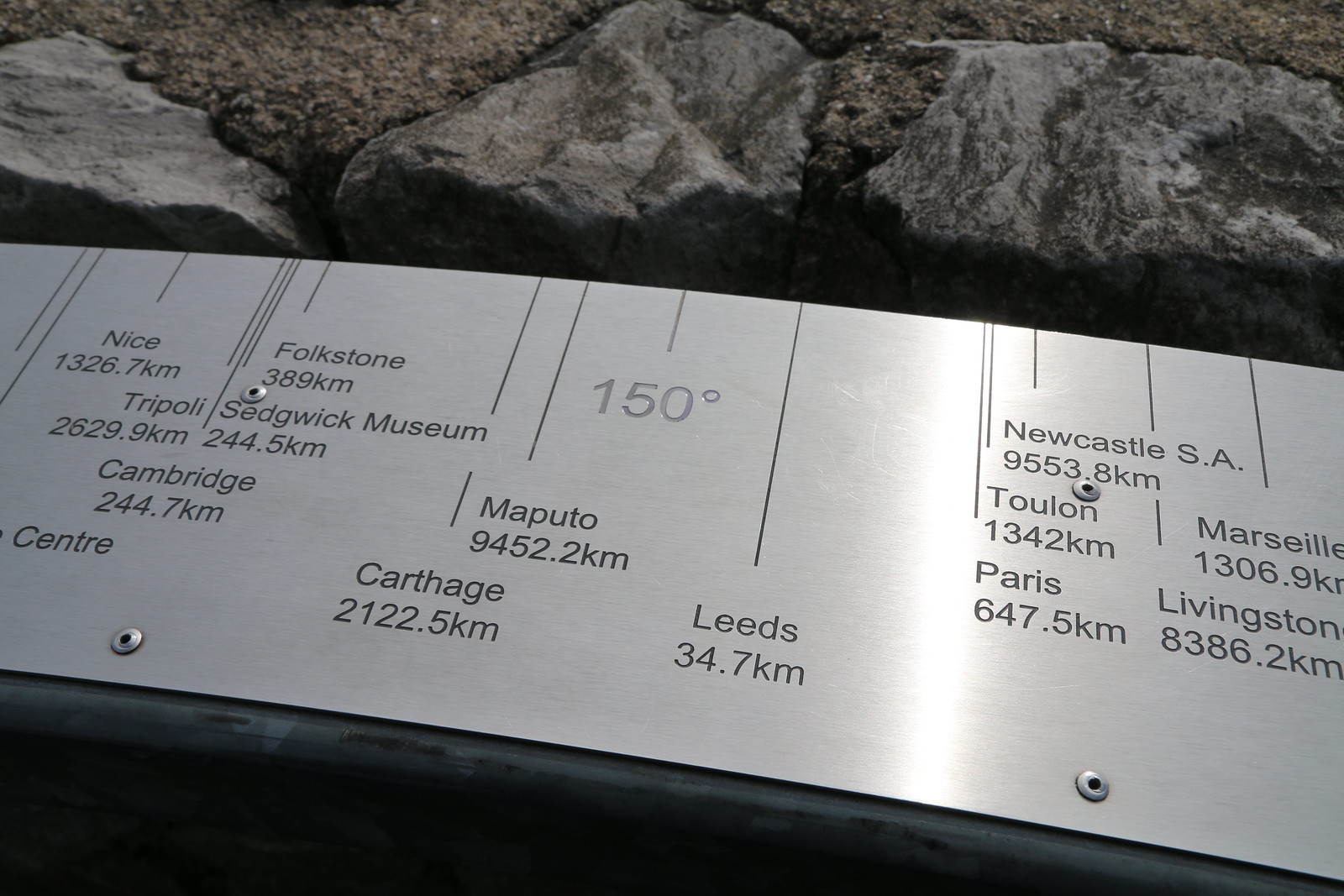This photo depicts a museum exhibit featuring a long steel measurement strip bolted securely into a rock formation, possibly part of a wall or the ground. Above the measurement device, large rocks are tightly packed, implying they cannot be easily removed. The metal strip is marked at the top with various lines resembling tick marks on a ruler, each line indicating the distance to different cities and landmarks in kilometers. For instance, it displays distances to Leeds (34.7 km), Paris (647.5 km), Nice (1326.7 km), Tripoli (2629.9 km), Cambridge (244.7 km), Sedgwick Museum (244.5 km), Folkestone (389 km), Carthage (2122.5 km), and Livingston (8386.2 km). Additionally, a line indicates an angle of 150 degrees. The exhibit appears to illustrate spatial relationships and distances between various global locations, all displayed on a steel plate set against a background of solid stone.